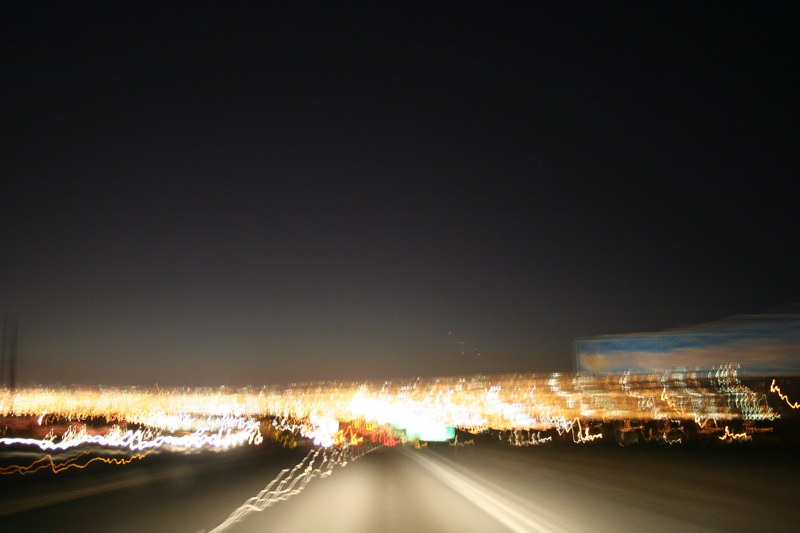This nighttime photograph appears to be taken from inside a moving car, capturing the blurred, dynamic scene of a highway beneath a dark, starless sky. The image is highly indistinct, likely due to motion, but it reveals a broad road ahead with a chaotic array of lights. These lights, predominantly white, orange, and yellow, stretch from the central point outward, resembling a city skyline illuminated at night. On the lower part of the photo, the bright, moving lights merge into a jumbled blur, suggesting motion. The right side of the image features a thick, blue, and pink light, possibly a part of a sign or building. Overall, the image conveys a sense of speed and night-time urban vibrancy, with no visible stars or moon in the horizon.